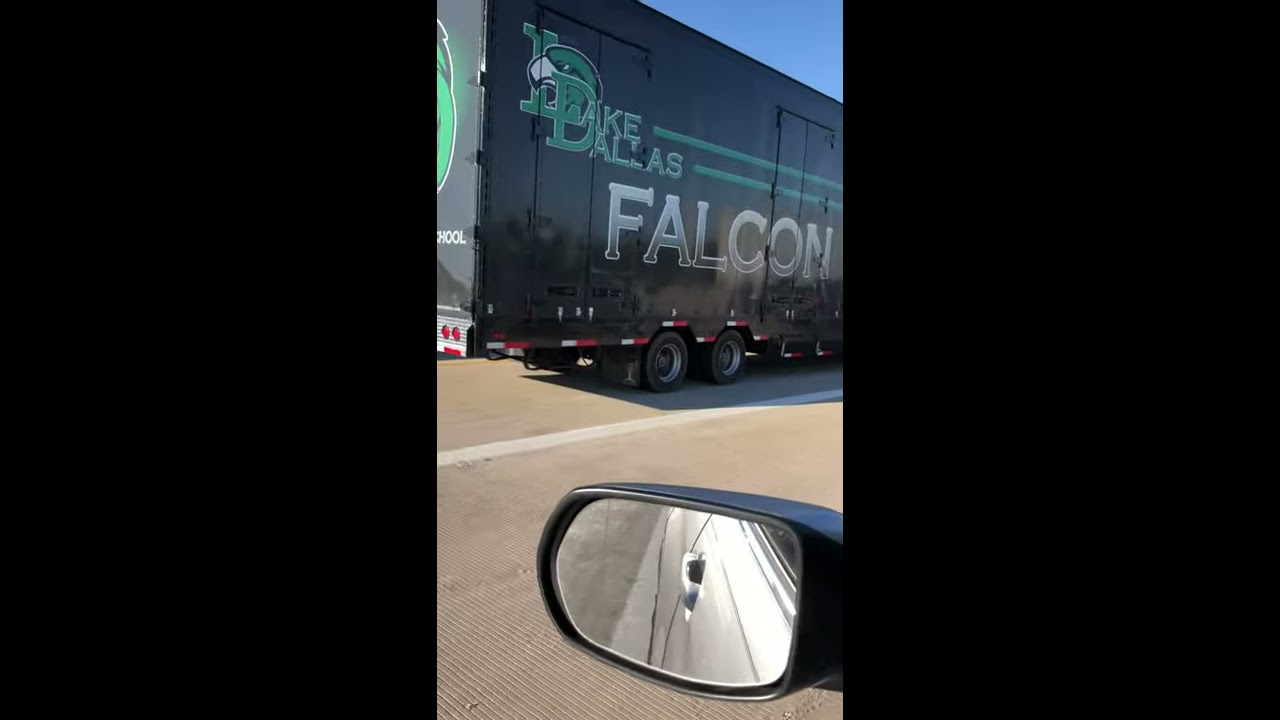The image depicts a large truck trailer, partially visible from the side and back, driving on a road, likely a freeway or interstate. The trailer is black with prominent green lettering at the top that reads "Lake Dallas," featuring a huge letter "D" and "L" alongside an eagle logo. Beneath this, in a gradient white-to-dark text, the word "Falcon" is displayed. The foreground includes the silvery exterior and the side view mirror of a car, indicating that the photo was taken from inside another vehicle. The truck's wheels and the lanes of the road provide additional context.